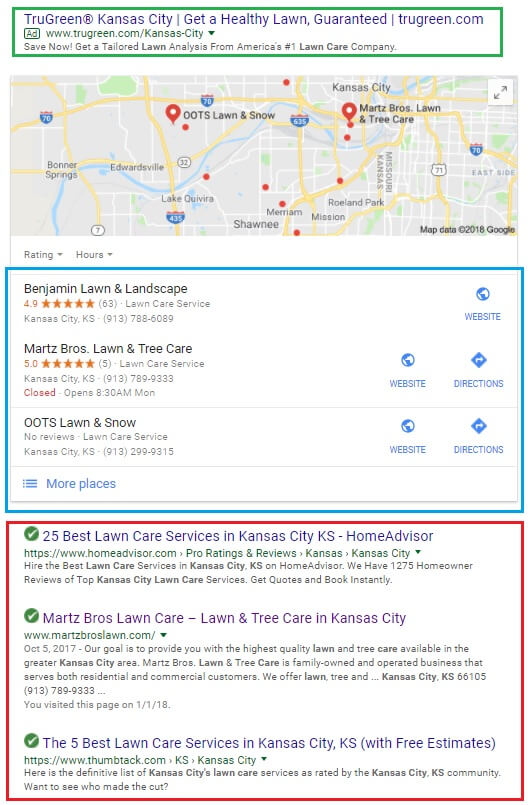"Experience the lush, vibrant green of a perfectly maintained lawn, brought to you by America's number one lawn care company, TruGreen. This image showcases a healthy and meticulously cared-for lawn in Kansas City, with rich soil and dense, emerald-green grass. TruGreen guarantees a beautiful and thriving lawn, ensuring your outdoor space remains pristine and inviting. Visit TruGreen.com for more information."